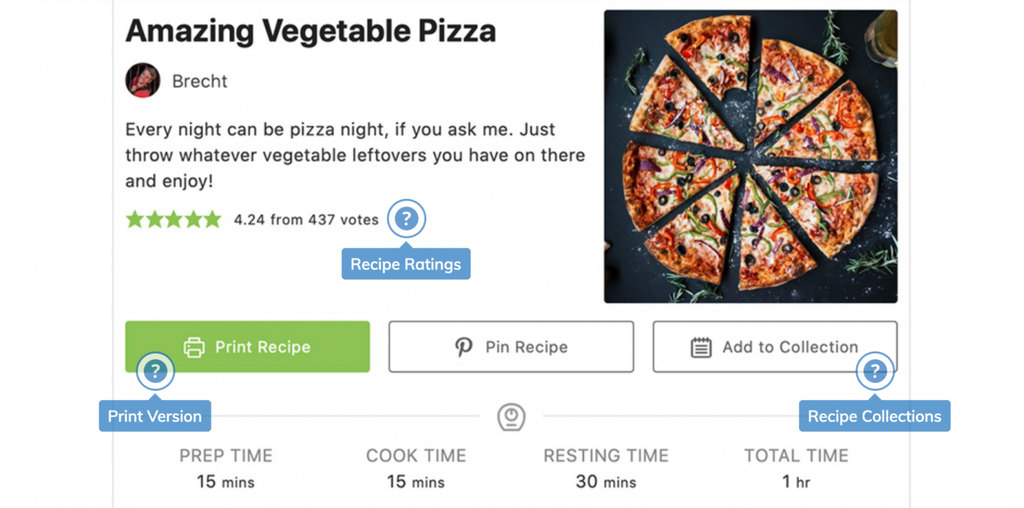This screenshot captures a recipe page viewed on a laptop or desktop screen. Dominating the upper left-hand corner in bold, large font is the recipe title: "Amazing Vegetable Pizza." The recipe is authored by Breck T., whose profile picture, displayed in a circular frame, shows an individual with short hair, though their gender is not easily discernible. Below the author's name, there's a brief summary that reads: "Every night can be pizza night. If you ask me, just throw whatever vegetable leftovers you have on there and enjoy."

The recipe's popularity is indicated by a rating of 4.24 stars out of 5, based on 437 votes. In the upper right-hand corner of the screen, there's a tantalizing image of the pizza, cut into eight slices with one slice having a bite taken out of it. Below this image, users are given the option to print the recipe, with the "Print Recipe" button highlighted in light green.